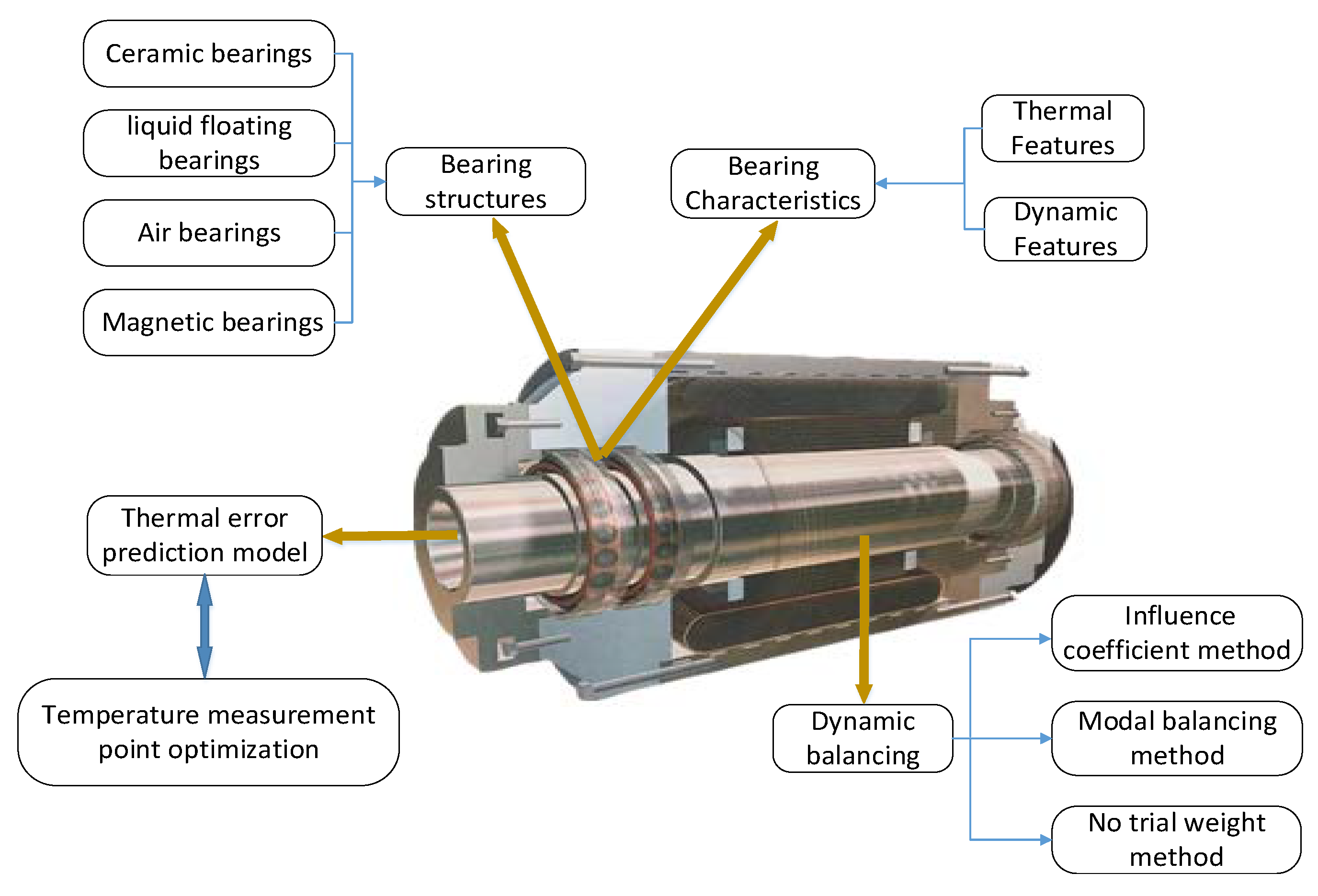The image is a detailed, color-coded diagram of a mechanical cylinder showcasing various bearings and their attributes. In the upper left, there are labeled blue boxes for ceramic bearings, liquid floating bearings, air bearings, and magnetic bearings, all connected by a blue line to "bearing structures." The center of the diagram features a 3D x-ray view of the interior of the cylindrical mechanism, likely a component of an engine or similar machinery, revealing its inner components. Surrounding this central image, many golden arrows point to white, curved rectangular word bubbles indicating different features and models, with black text labels. On the bottom left, there's a section dedicated to thermal error prediction, which includes models and temperature measurement points for optimization. Also, in this area, yellow arrows highlight thermal features and dynamic features, all connecting to bearing characteristics. In the bottom right, several methodologies are listed, such as the influence coefficient method, model balancing method, no trial weight method, and dynamic balancing. The entire image uses detailed labeling and color-coded arrows to explain the intricate relationships and characteristics of the mechanical components.